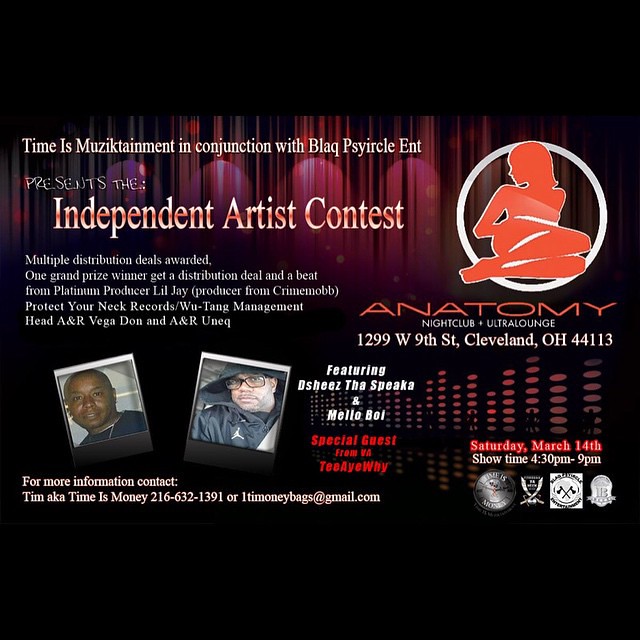The flyer advertises an Independent Artist Contest taking place at the Anatomy Nightclub and Ultra Lounge, located at 1299 West 9th Street, Cleveland, Ohio, 44113, on Saturday, March 14th, from 4:30 PM to 9:00 PM. The backdrop of the flyer is stark black with maroon curtains, presenting a professional yet dramatic aesthetic that draws attention. 

The upper right corner features the club's logo: a white circle showcasing a red silhouette of a woman laying down. The text on the flyer highlights multiple distribution deals to be awarded, with the grand prize winner receiving a distribution deal and a beat from platinum producer Lil' J, known for his work with Crime Mob and Protect Your Neck Records under Wu-Tang Management Head, A&R. 

Prominent attendees include Deshies, The Speakah, and Mellow Boy, with special guest T-A-Y from Virginia. Pictures of two young men paying homage to the event are displayed towards the left side of the flyer. 

The event is presented by Time is Music Tainment in conjunction with BL AK Cyrical Entertainment. For additional details, contact Tim, a.k.a. Timeismoney, at 216-632-1391 or via email at onetimmoneybags@gmail.com. The flyer integrates a color palette of red, orange, purple, white, gray, brown, black, and gold to enhance its visual appeal and readability.